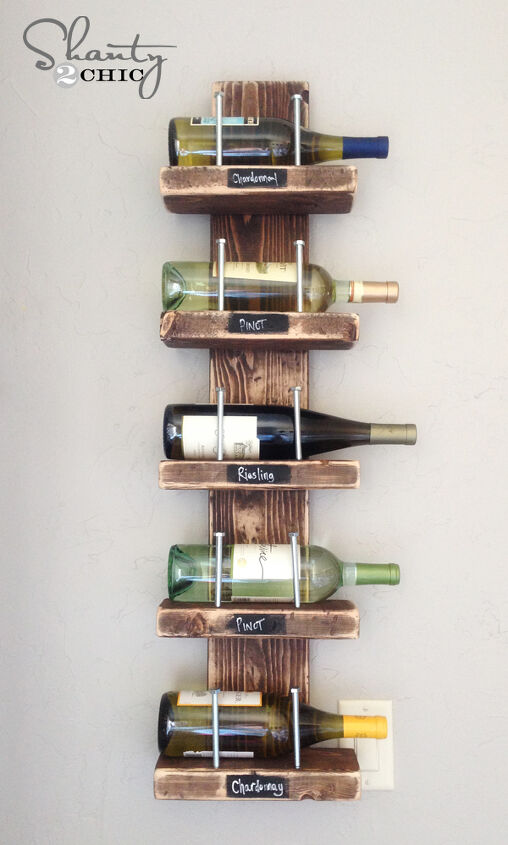In this tall, vertically oriented photograph, we see a stylish and functional wine rack mounted on a light tan or off-white painted wall. The wine holder, branded with the logo "Shanty Too Chic" written in elegant gray cursive at the upper left, is fashioned from a medium-toned 2x4 wooden plank with five short shelves attached. Each shelf is designed to hold one wine bottle securely, reinforced with two long vertical bolts at the front to prevent the bottles from rolling off. The shelves feature rectangles of black chalkboard paint on the front, with each bottle labeled in white: from top to bottom, Chardonnay, Pinot, Riesling, Pinot, and Chardonnay. The minimalist yet effective design creates a practical and eye-catching display for any wine enthusiast.